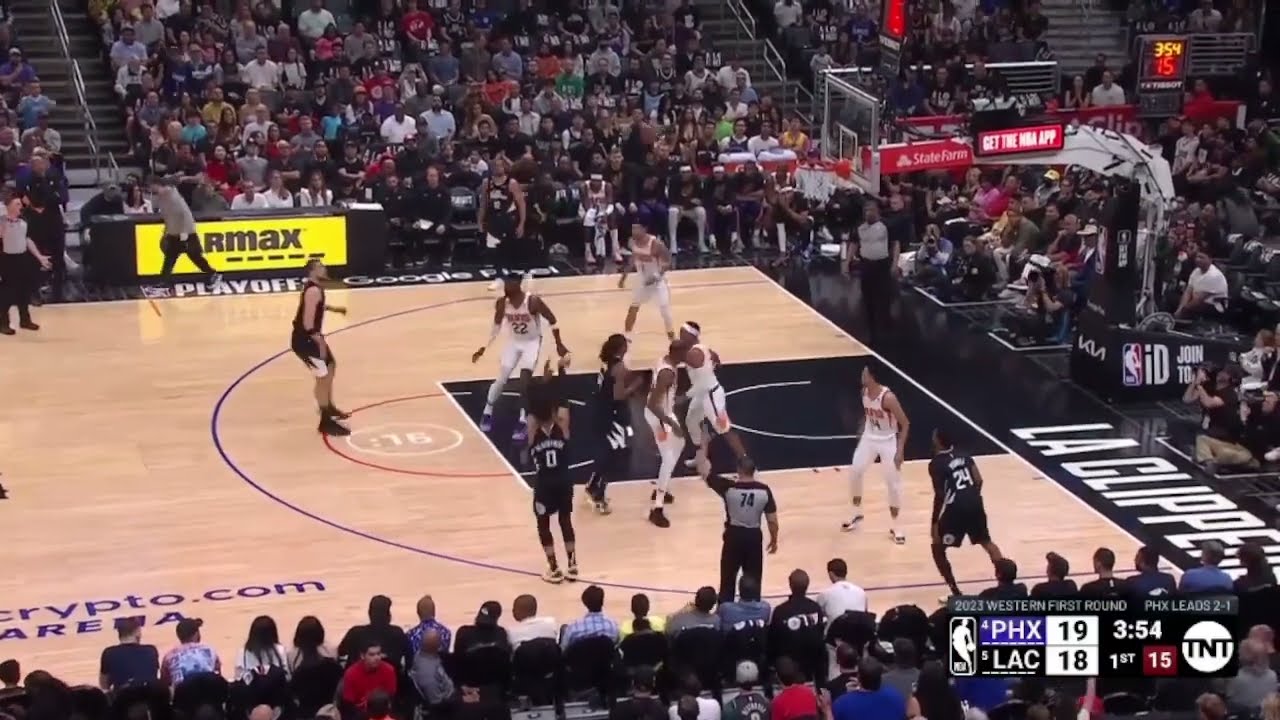The image is a wide rectangular screenshot capturing a live professional basketball game between the Phoenix Suns (PHX) and the LA Clippers (LAC). The view is slightly diagonal, showcasing a dynamic play unfolding toward the basket located in the top right corner. Five players in white uniforms, representing PHX, are on defense while five players in black uniforms, representing LAC, are on offense. The game takes place in a packed arena with a large crowd visible both at the top and bottom sections of the image.

The basketball court features clearly defined lines, including the three-point line, on a light tan surface surrounded by black. The scoreboard in the bottom right corner indicates a score of 19-18 in favor of Phoenix, with 3:54 left in the first quarter. The score display also includes the PHX abbreviation in purple and LAC in black, with the game broadcasted by TNT, whose logo appears alongside the score. Notable on-court markings include "crypto.com arena" and an advertisement for Miramax.